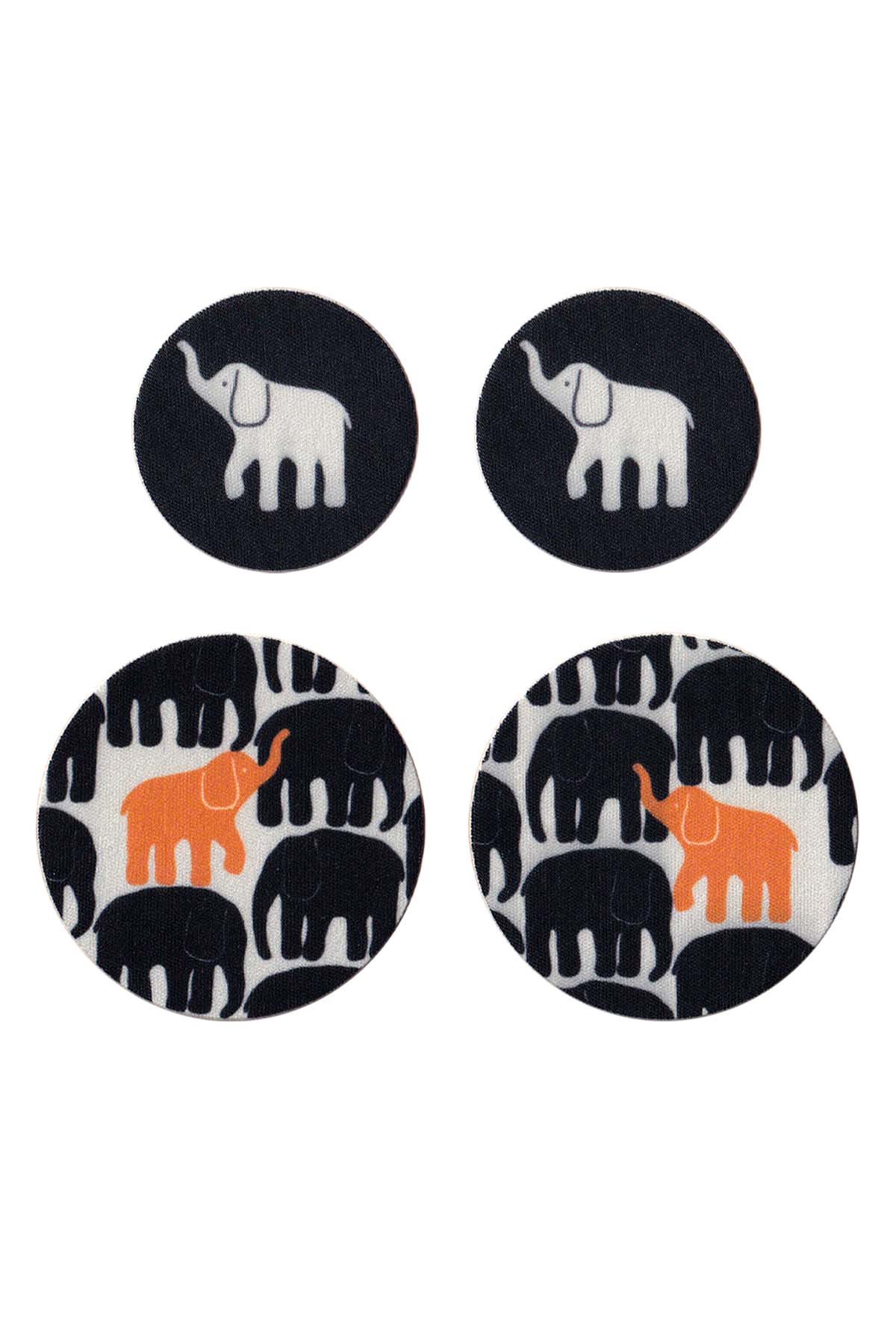This image features four circular artworks arranged in a grid, with two on top and two on the bottom. Each artwork revolves around an elephant theme, with distinct differences in style and color.

The top left circle showcases a simple outline of a white elephant, with its trunk raised and its right front leg lifted, facing left against a black background. Its counterpart on the top right mirrors these exact features, including the elephant's pose and black background.

On the bottom left, the larger circle displays multiple blue elephants on a white background, with one unique orange elephant that stands out among them. This orange elephant faces a distinct direction compared to the others. The bottom right circle mirrors the bottom left, also featuring numerous blue elephants on a white background, with the standout orange elephant oriented differently than in the left circle.

Overall, the top pair of artworks mirror each other with a consistent design, while the bottom pair reflect a mirrored pattern with an emphasis on the contrasting orange elephant.